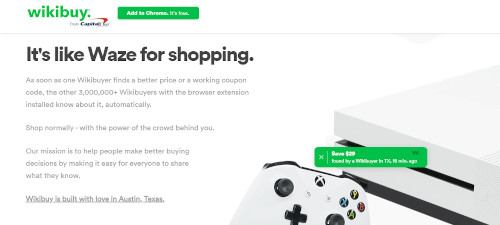Here is the cleaned-up, detailed caption:

---

The image primarily showcases a minimalist design with a white background, interspersed with green, black, and gray text. In the upper left corner, the green text reads "Wikibuy" and below it, in smaller black text, it says "From Capital One." Adjacent to this is a green button that appears to say "Add to Chrome" — although the resolution makes it somewhat unclear, it is implied that the extension is free.

Below this, a sentence in black text reads, "It's like Waze for shopping. As soon as one Wikibuyer finds a better price or a working coupon code, the other three million plus Wikibuyers with the browser extension installed know about it automatically. Shop normally with the power of the crowd behind you. Our mission is to help people make better buying decisions by making it easy for everyone to share what they know. Wikibuy is built with love in Austin, Texas."

To the right, there is an image of an Xbox One console system accompanied by a white controller. The controller features black joysticks, buttons, and bumpers, along with colored buttons marked Y (yellow), B (red), A (green), and X (blue). The console itself features a white and black color scheme. Below this, there is a green button displaying a price, followed by text that seems to mention Wikibuy in Texas, though the low resolution makes it difficult to decipher.

---